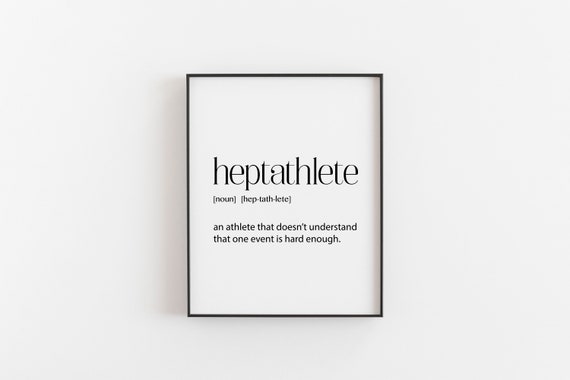The image is a color photograph showcasing a minimalist piece of wall art. It features a simple black industrial-style frame, proportioned like an 8.5 by 11 sheet of paper, hung against a white background. The frame encloses a white piece of paper with black text. Centered and in large, bold lowercase letters, the word "heptathlete" is displayed. Beneath this, in much smaller text, it reads "noun, heptathlete," with the phonetic pronunciation. Further below, in even smaller black text, the definition "an athlete that doesn't understand that one event is hard enough." A very slight shadow is cast to the left side of the frame, emphasizing its presence on the white wall.